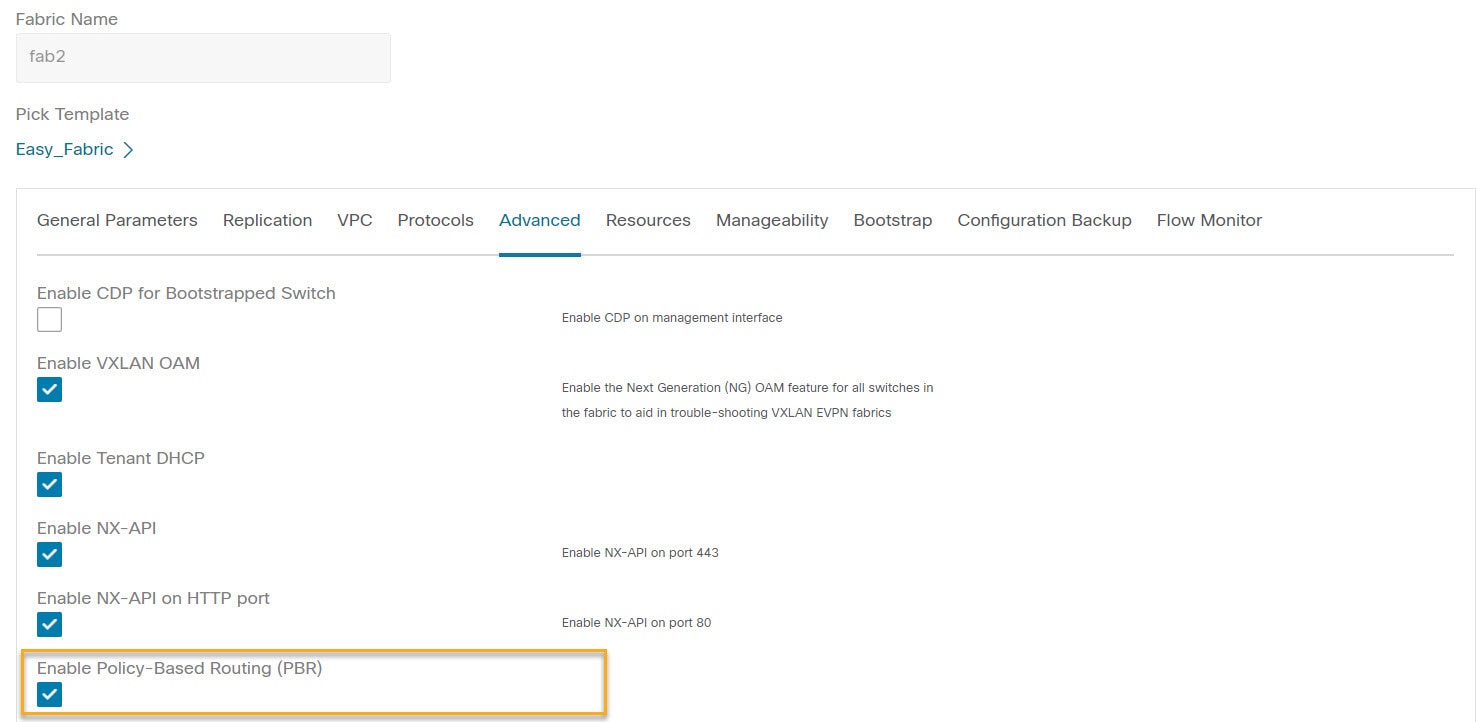This screenshot captures a partially visible section of a web interface, predominantly showcasing text over a minimalist design. The interface features a basic black text on a white background layout, with minimalistic use of blue for radio buttons and highlighted text, adding some visual contrast.

At the very top left corner, there's a text input labeled "Fabric Name," where "Fab 2" has been entered as the text value. Below this, an option to pick a template is visible, with "Easy_Fabric" being the currently selected template.

The top toolbar presents a comprehensive list of navigational options including:
- General Parameters
- Replication
- VPC Protocols
- Advanced Resources (the currently selected option)
- Manageability
- Bootstrap
- Configuration Backup
- Flow Monitor

Under the "Advanced Resources" section, a detailed view of selectable options with radio buttons is displayed. Among these, the option marked with a yellow rectangle, likely added for instructional purposes in the screenshot, is "Enable Policy-Based Routing (PBR)."

The screenshot's purpose seems to be to guide someone through enabling Policy-Based Routing (PBR) within the "Advanced Resources" settings. Unfortunately, due to the cutoff nature of the screenshot, critical identifying information about the website, such as company name or specific taglines, is missing, leaving the exact source unclear.